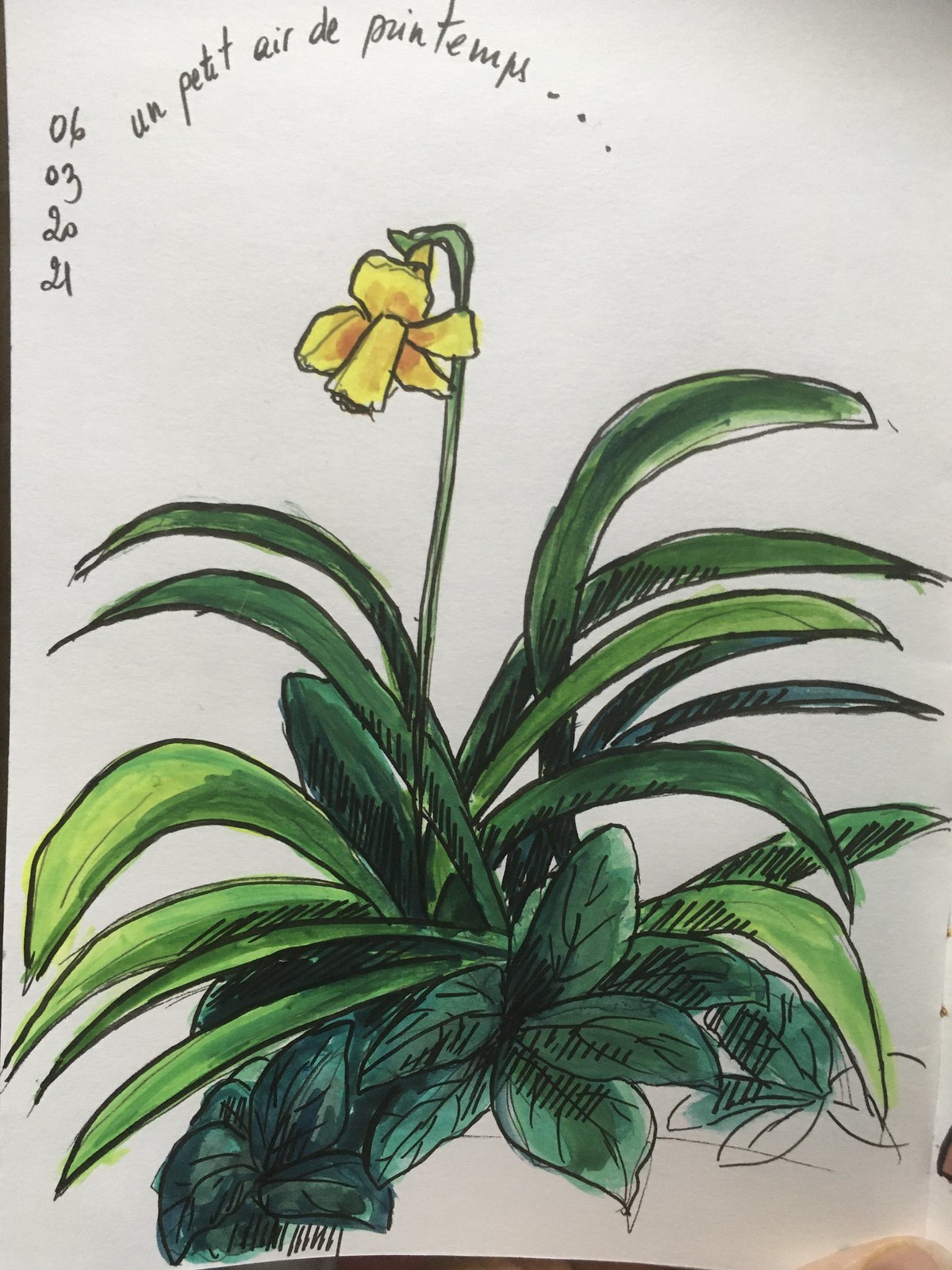This detailed sketch, done on white paper with an intricate black ink outline and colored with vibrant markers, features a central plant with a single, tall green stem supporting a drooping yellow flower. The plant's base is adorned with various leaves, combining round, oval-shaped dark green leaves and pointy, lime green to jade-colored leaves. These elements suggest a careful contrast in colors and shapes, creating a dynamic botanical composition reminiscent of an iris. In the top left corner, elegant French handwriting in a clean script font reads, "Un Petit Air des Printemps," adding a touch of sophistication. Nearby, the numbers "06, 03, 20, 21" are inscribed, although their significance remains unclear. The overall effect is a harmonious blend of colors and textures that evoke the freshness of spring.